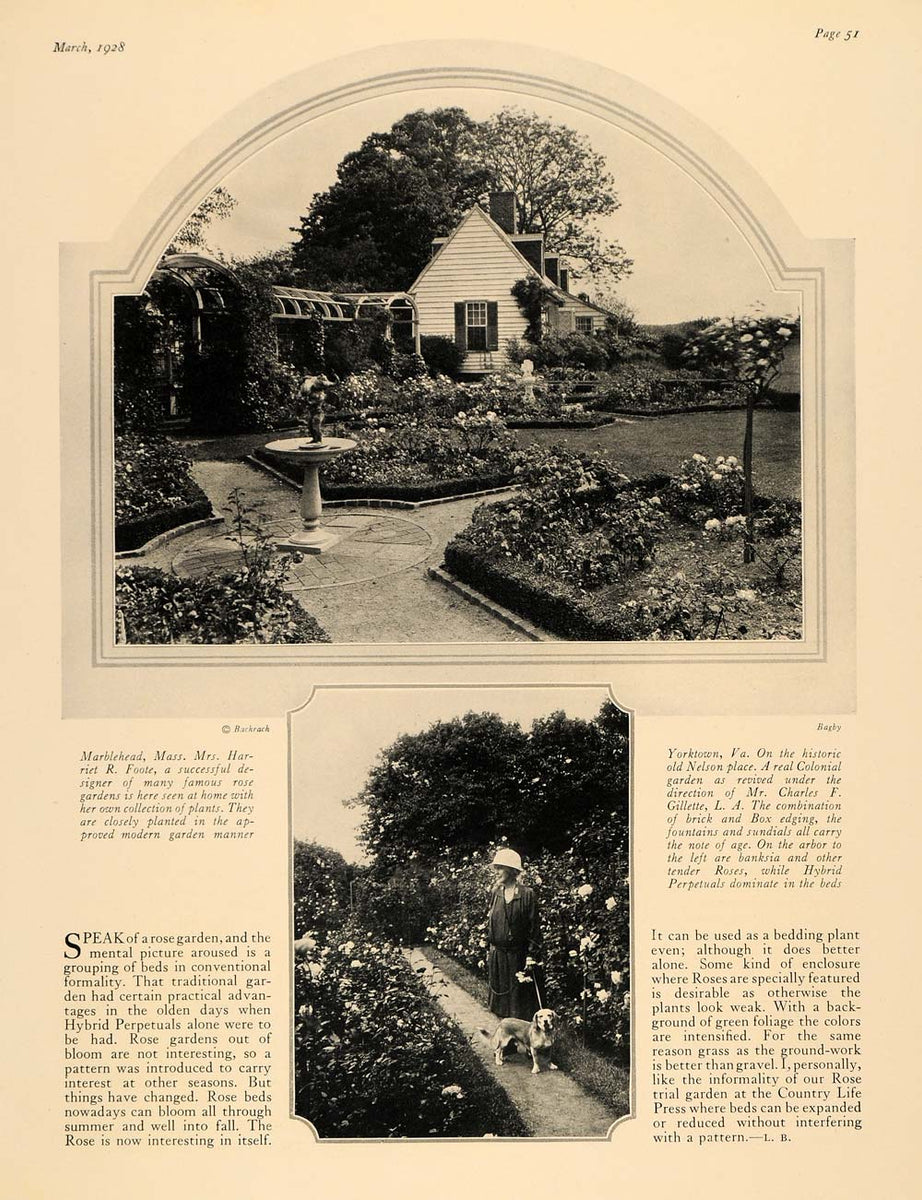This scanned page from a 1928 publication, marked as March 1928, on page 51, features a black and white photograph of a beautifully landscaped front yard. The garden, designed by the accomplished Miss Harriet R. Foote, includes a central birdbath surrounded by intersecting tiled or stone paths that divide the area into four sections filled with lush bushes, likely roses. Behind this picturesque garden stands a single-story, elegant house, which is presumably in Yorktown, Virginia. An additional smaller image at the bottom of the page depicts Miss Foote herself, dressed in 1920s attire with a white hat, accompanied by her dog as they stroll through the garden's meticulously planted rose aisles. The accompanying text, appearing in paragraphs to the left and right of the photograph, discusses Miss Foote's success as a rose garden designer and provides more details about the exquisite garden's layout.